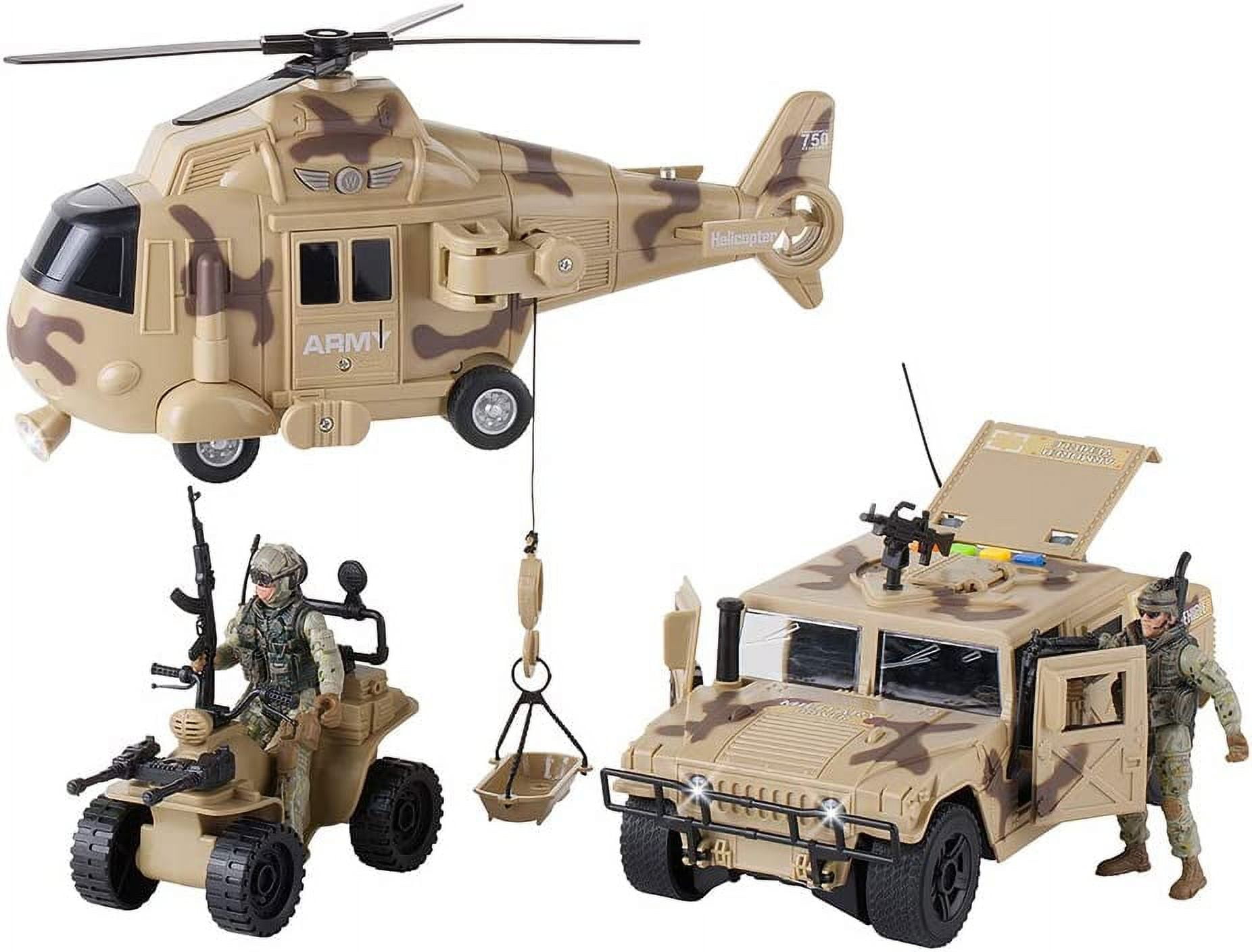The image depicts three detailed Army-themed toys against a white background. In the top left corner, there's a brown camouflage helicopter marked with "750" on the rear wing and "helicopter" below it. It features two black landing wheels, black main rotors, and fenestron tail rotor. The body of the helicopter has darker brown patches, and on the side door, it reads "army" in white letters. Additionally, the helicopter has a wire with a basket on the left side. On the bottom left, there's a soldier riding a beige and black ATV. The soldier is equipped with a helmet and appears to be holding a rifle, with additional guns mounted on the front of the vehicle. In the bottom right corner, the image shows a brown camouflage Humvee with an open door and rear hatch. The Humvee is fitted with an M60 gun on top and a soldier standing adjacent to it. Each toy features intricate details suitable for children around five years old, showcasing realistic military gear and vehicle designs.